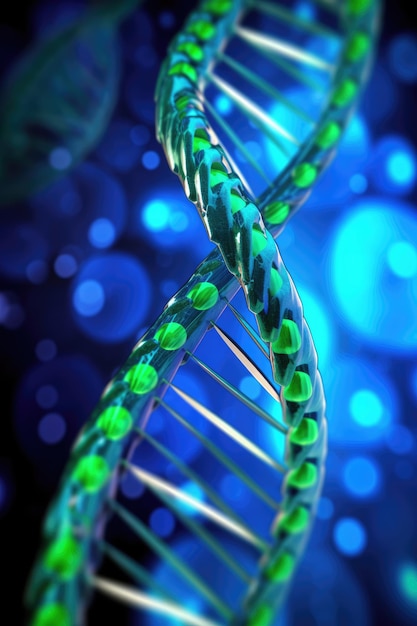The image is a vertical rectangular illustration, featuring a detailed DNA double helix in the foreground. The background is a gradient of dark blue on the left, transitioning to a lighter blue on the right, creating a sense of depth. Scattered across this backdrop are variously sized blue circles, resembling out-of-focus lights or bubbles, adding a modern and dynamic visual texture. Central to the image are two twisting, transparent DNA strands with white rungs connecting the sides, mimicking a twisted ladder. Interspersed along the helix are small green dots, adding vibrant details. The DNA’s structure and green dots stand out sharply against the consistent blue circles of the background, which seamlessly continues behind the DNA, enhancing the three-dimensional effect.